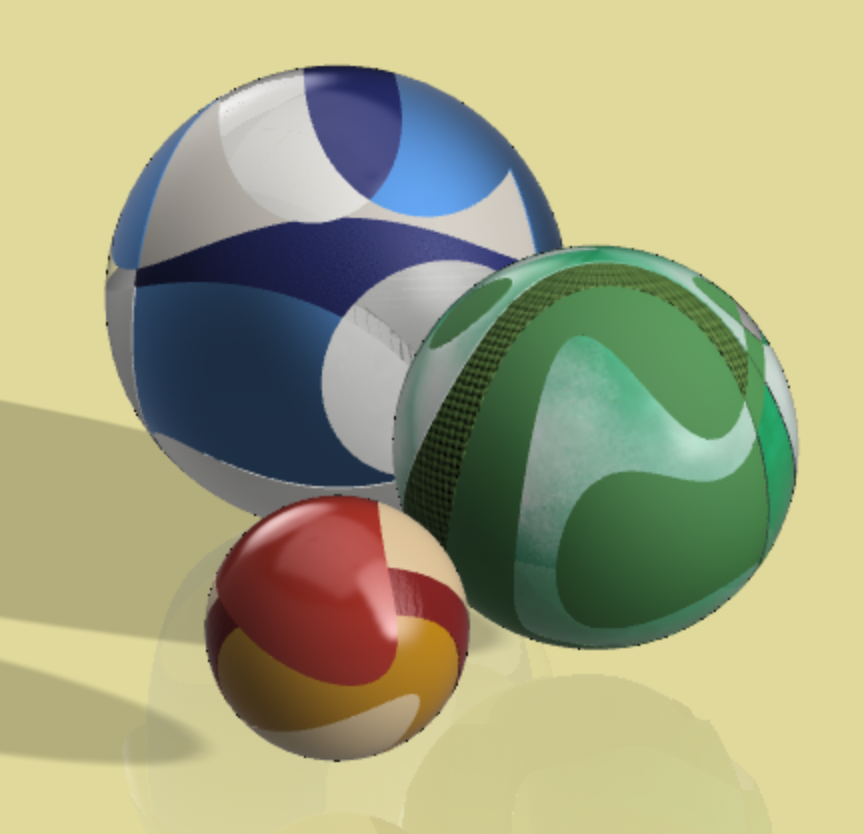The image depicts three intricately designed balls set against a light beige-yellow background. The largest ball, positioned from the upper left to the center, is predominantly blue with a variety of patterns including white, gray, navy blue, and lighter blue, resembling fishtails and circles. The medium-sized middle ball, located slightly in front and to the right of the blue ball, features swirly patterns in different shades of green, such as shiny light green, matte dark green, and a dark checkered green. The smallest ball, situated in the front and mostly in the lower left, boasts a design with swirls and bands in cream, red, yellow, and tan. The balls appear to cast shadows, suggesting a light source, but the image overall seems to be a computer-generated artwork or painting, with a slightly pixelated texture indicating low-resolution or deliberate artistic rendering.